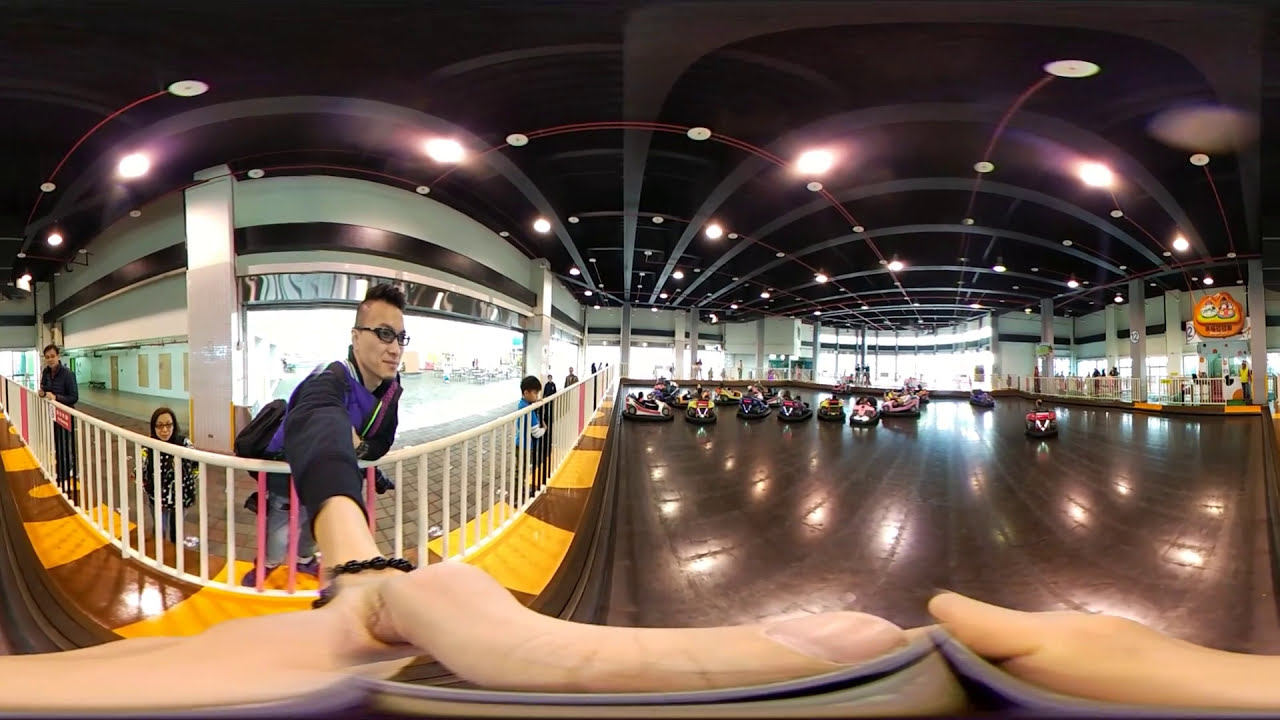In this vibrant indoor scene, we are inside a spacious building with a high ceiling adorned with numerous lights, whose reflections shimmer on the laminated wooden floor below. The focal point is a captivating glimpse of a go-kart or bumper car track for kids, filled with small colorful vehicles—red, pink, yellow, and blue—scattered across the shiny surface. A man with glasses, sporting a black long-sleeved shirt and a black bracelet on his right wrist, leans over the railing on the left side, holding up what appears to be a GoPro wide-angled camera. His distinctive Mohawk hairstyle adds to his noticeable presence. To his right, a woman wearing spectacles and a coat with yellow stripes is crouched down, also observing the lively scene. The track area is spacious, with a large open section at the far end allowing sunlight to stream through, creating a luminous atmosphere. Behind the man, there are a couple of kids standing, attentively watching the fun-filled action on the track. The entire image seems to be captured as part of a 360° panorama, adding a dynamic and immersive perspective to the bustling indoor playground.